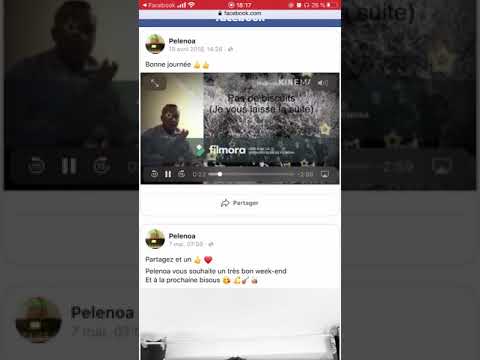The image is a low-resolution screenshot of someone's Facebook feed, captured from a phone, indicated by the red bar at the top displaying signal status and other phone indicators. Below the red bar, there's a white bar with "Facebook.com" in blue font, reinforcing that this is indeed Facebook. The main part of the feed shows a post by someone named Polonoa, who has written "Bonne Journée" accompanied by two thumbs-up emojis, indicating a French greeting. The post prominently features a video thumbnail of a person staring forward and to the right, surrounded by various plants, and adorned with the watermark "Filmora." Beneath the main post, there are additional elements, including more text and commonly seen Facebook emojis like thumbs-up and heart, amidst some more French writing. The image is notably blurry, making some details and numbers indiscernible.